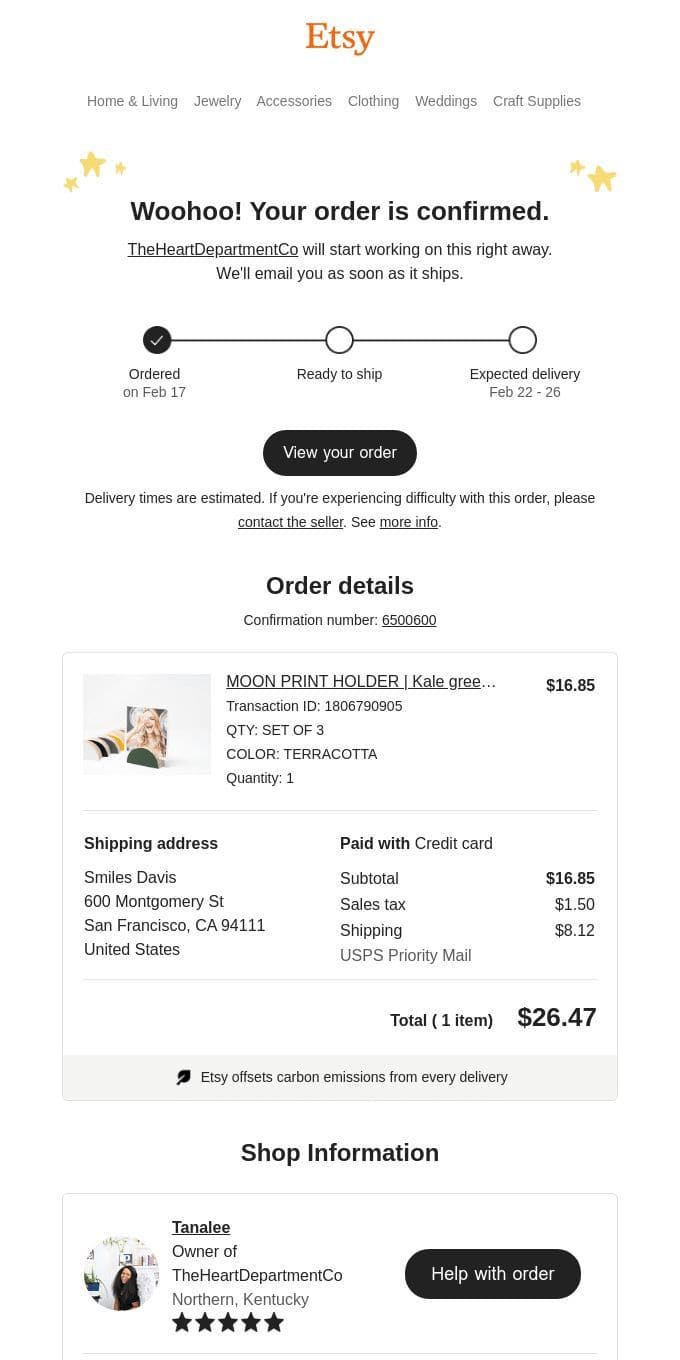The image displays an order confirmation page from Etsy. At the top, "Etsy" is prominently written in orange letters on a white background. Below this, category links are listed: "Home and Living," "Jewelry," "Accessories," "Clothing," "Weddings," and "Craft Supplies." Gold stars accompany a celebratory message: "Woohoo, your order is confirmed. The HART Department will start working on this right away. We'll email you as soon as it ships."

Moving down, a black circle with a checkmark indicates, "Ordered on February 17th." A line connects this to another white circle labeled, "Ready to ship," which further connects to another white circle stating, "Expected delivery February 22nd through 28th."

Beneath this, a black box with white text invites the user to "View your order." Further details include: "Order details, Confirmation number" (too small to read). The ordered item, "Moon print holder," is listed at $16.85 with a quantity of three in terracotta color. Payment method is specified as credit card, with a subtotal of $16.85, sales tax amounting to $1.50, shipping cost of $8.12 via USPS priority mail, culminating in a total of $26.47 for one item.